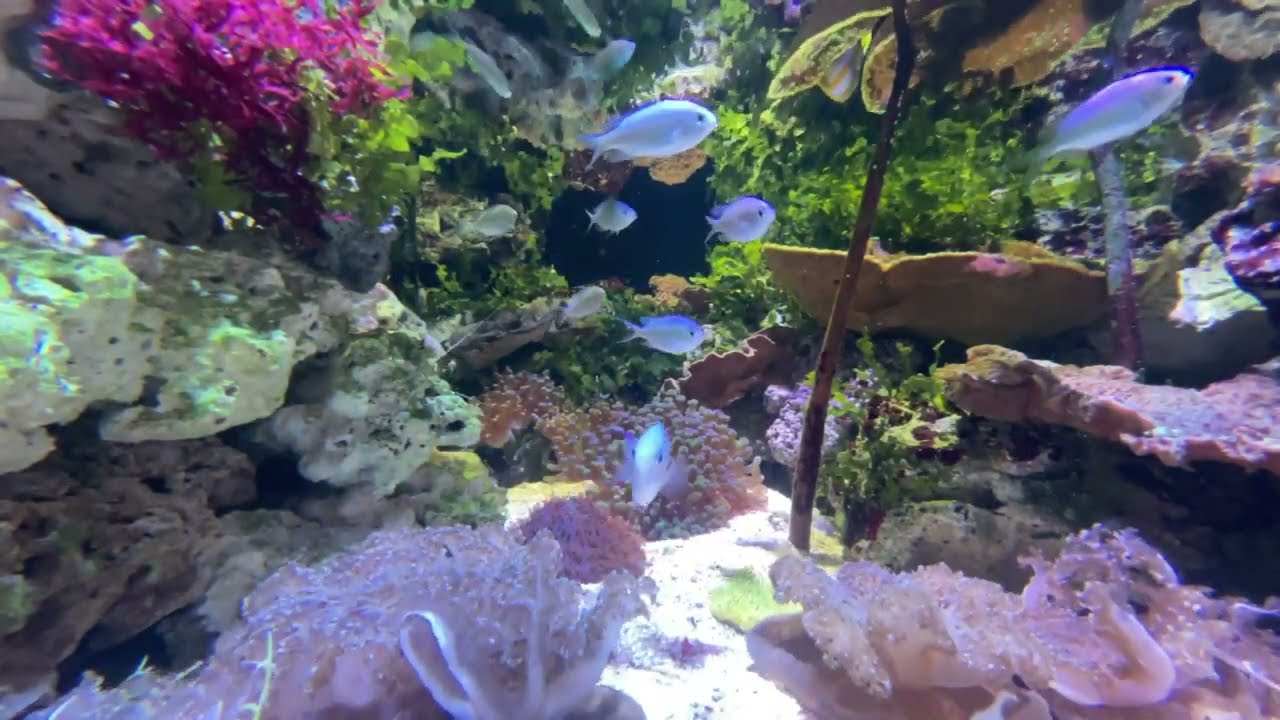The image captures a vibrant underwater scene, likely taken in a large aquarium or the ocean. Bathed in sunlight from above, the seabed is covered with white sand and various richly colored coral and rocks. On either side of the image, there are textured rock formations with green seaweed and moss. The left side features a striking mix of a reddish-pink plant intermingled with bright green vegetation, blending into the rocky surface. The right side showcases a tiered arrangement of rocky ledges also adorned with green plants. Meanwhile, the upper left corner holds a patch of purplish vegetation adding to the saturated hues. Silvery blue fish, resembling tiny silver dollars, are scattered throughout the scene, swimming serenely. The center of the image offers a clear view into the darker depths, highlighting the crispness and clarity of the underwater tableau.